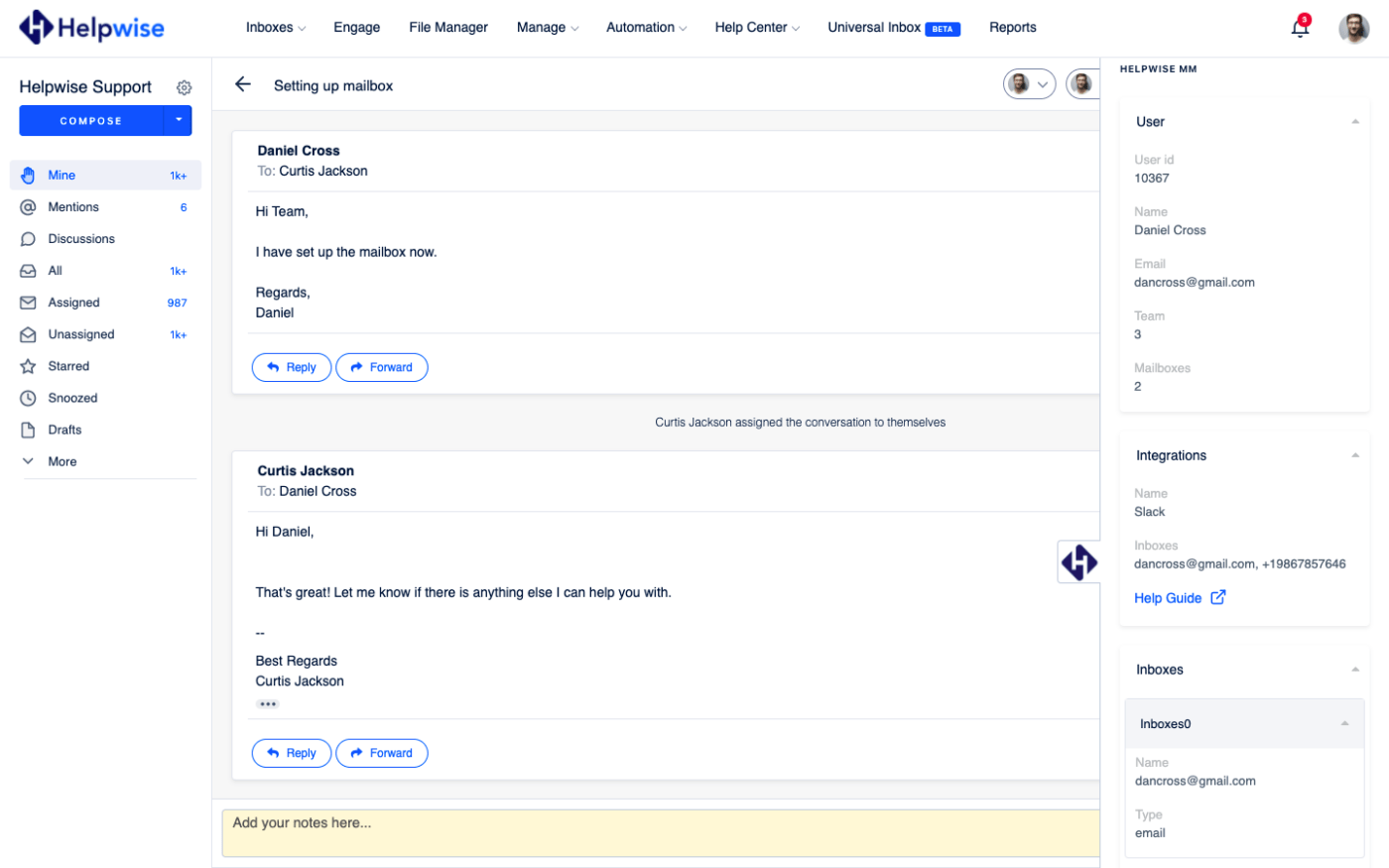A screen capture of the Helpwise dashboard is showcased. The Helpwise logo prominently sits at the top left, resembling a blue yield sign shaped like a diamond with an extended H in the center, featuring darker navy blue for "Help" and light blue for "wise." The top menu bar includes tabs labeled: Inboxes, Engage, File Manager, Manage, Automation, Help Center, Universal Inbox (beta), and Reports. On the far right, there are notification icons and a user profile icon.

To the left, a "Helpwise Support" section is visible. Below it are clickable options such as "All" (highlighted in blue) and "Mine" (in light gray), followed by a series of other menu items.

On the main screen, an email thread is shown. At the top of the thread, "Daniel Cross to Curtis Jackson" is noted, with "Daniel Cross" in bold and "Curtis Jackson" in light gray. The message from Daniel reads: "Hi team, I have set up the mailbox now. Regards, Daniel." Below, there are options to Reply or Forward the message.

Further down, a response from "Curtis Jackson to Daniel Cross" is displayed, with "Curtis Jackson" in bold. The message states: "Hi Daniel, that's great. Let me know if there's anything else I can help you with. Best regards, Curtis Jackson." At the bottom, there is a section to add notes.

Overall, the image provides a comprehensive view of the Helpwise interface, highlighting its design, sections, and functionalities.